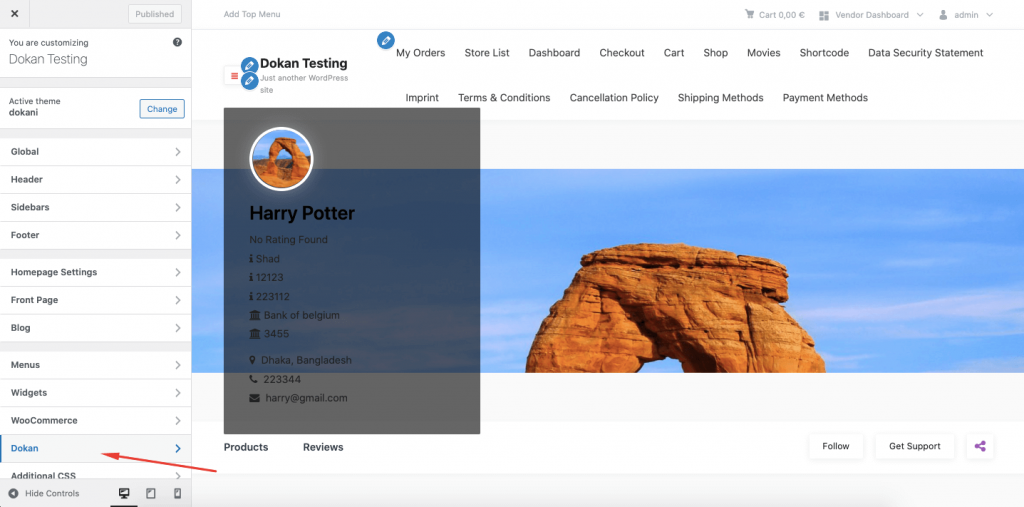Here is the cleaned-up and detailed caption:

"A cropped screenshot taken from a web-based application, likely a website-building tool, showcases the interface of the software. The left-hand side menu features various navigation options, including Global, Headers, Sidebars, Footer, Homepage Settings, Front Page, Blog, Menus, Widgets, Blue, Commerce, and Dokkan. The 'Dokkan' option is highlighted in blue, accompanied by a red arrow pointing to it. The main section of the screen displays a preview of a website titled 'Dokkan Testing,' featuring an e-commerce-style layout suggesting it is an online shopping platform."